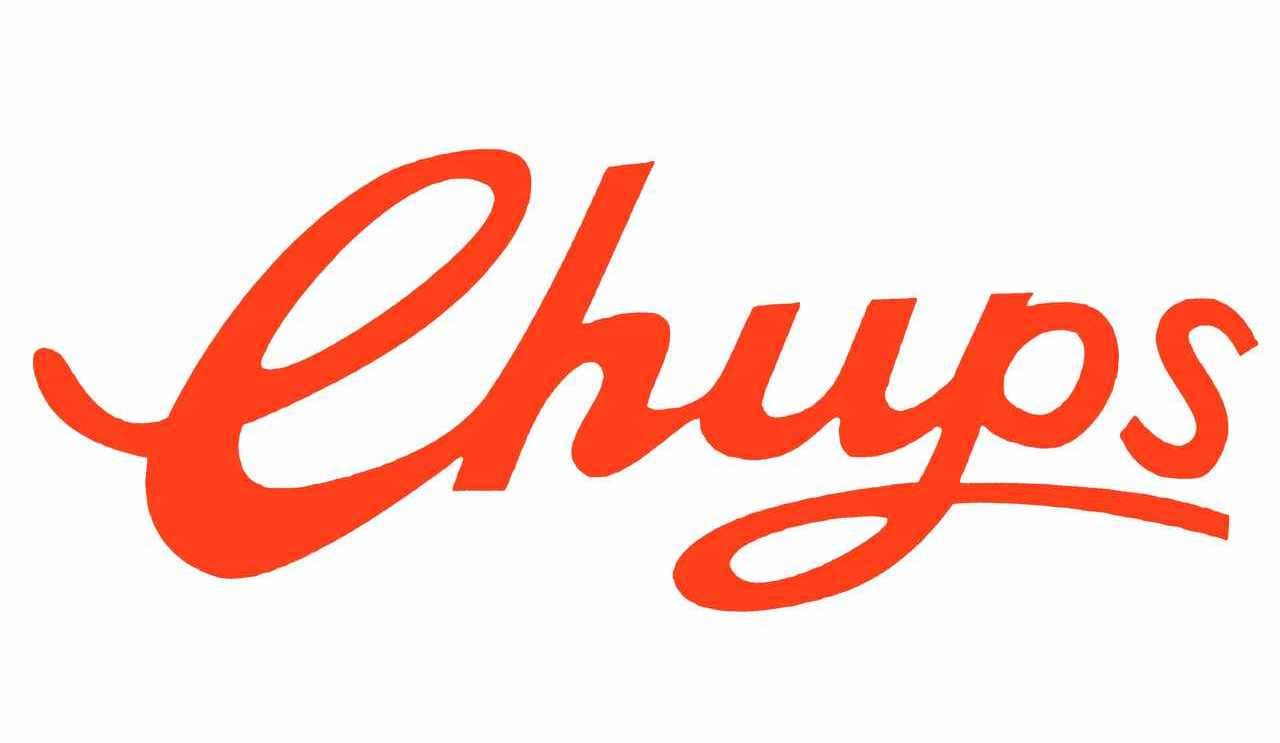This image features a stylized segment of the Chupa Chups logo, particularly highlighting the red, cursive text "CHUPS" against a pristine white background. The lettering is a vivid red, with subtle variations suggesting a darker red outline. Noteworthy aspects include the intricate curls in the capital 'C' and the sizeable swirl beneath the 'P,' which also serves to underline the 'S.' The entire text forms a flowing, interconnected cursive script, with the exception of the 'S,' which stands apart as a regular lowercase letter. Additionally, the text arrangement shows a slight curvature, dipping gently towards the ends and rising slightly in the middle. The image appears to contain compression artifacts around the lettering, hinting that the graphic might have been saved from a higher quality source at some point.